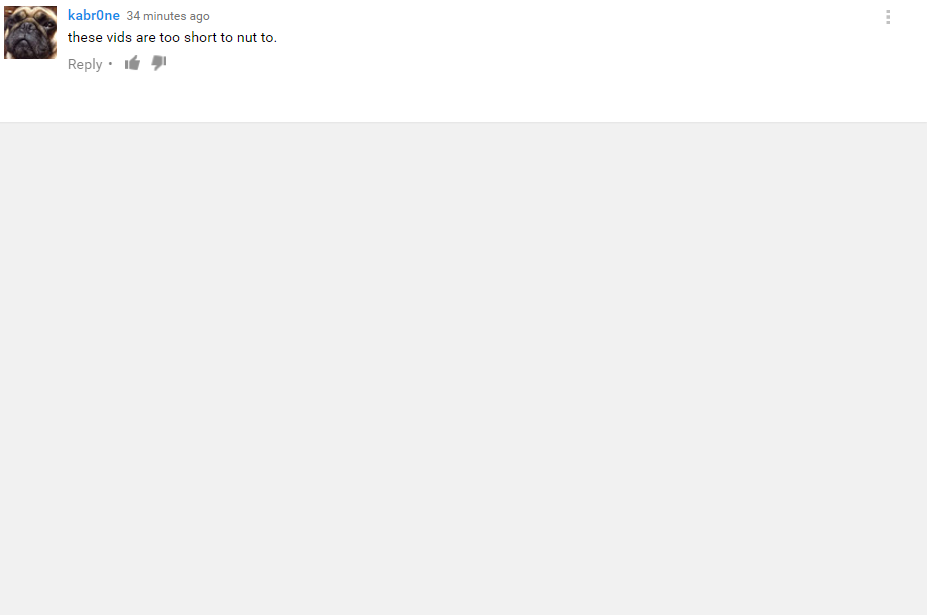The image is a screen capture of a single social media post, potentially from Twitter or a similar platform. The user's avatar is a square-shaped image of a pug with a wrinkly face. The dog has large, expressive black eyes looking upward; the top of its head is brown, while the area around its eyes and snout is black. 

The username of the person who posted is "Kabroné," with the handle spelled as K-A-B-R-0-N-E, using a zero instead of the letter "o." The post was made 34 minutes ago. The content of the post reads, "These vids are too short to not." 

Below the post, there are options to reply, indicated by the word "reply," followed by a dot, and icons resembling a thumbs up and thumbs down, which are in gray silhouette. The background of the screen capture is white, and in the top right corner, there is a vertical ellipsis (three dots arranged vertically), possibly indicating additional settings or options.